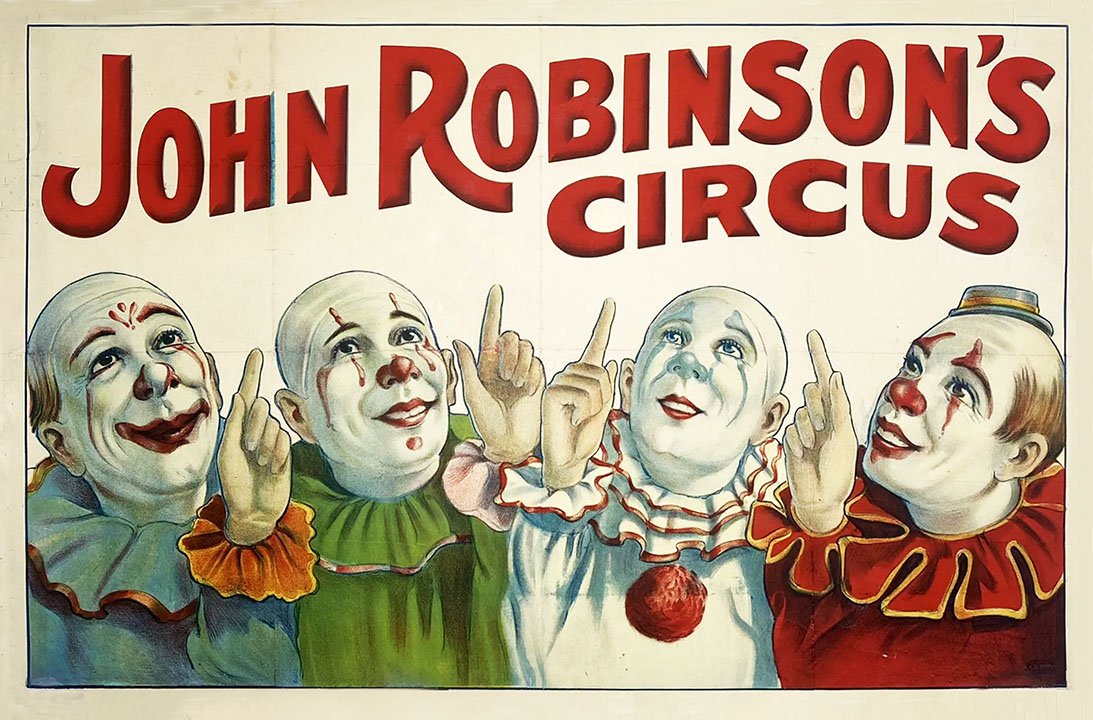This image is a horizontal, vintage-style circus poster with a thin black border. It prominently features large, red beveled text at the top that reads "John Robinson Circus", with a subtle wave-like flow to the letters. Below the text, there are illustrations of four clowns, each with white face paint, red lips, and both red and white noses, pointing up towards the text. From left to right, the first clown wears a blue suit with an orange trim on the hand, the second wears a green suit with a pinkish trim on his open-collared sleeve, the third dons a white and red suit with a white and red trim, and the fourth clown is dressed in a red suit with a gold trim and a comically small blue and gold hat. The entire scene is set against a white background, encapsulating a whimsical and nostalgic feel of the circus.